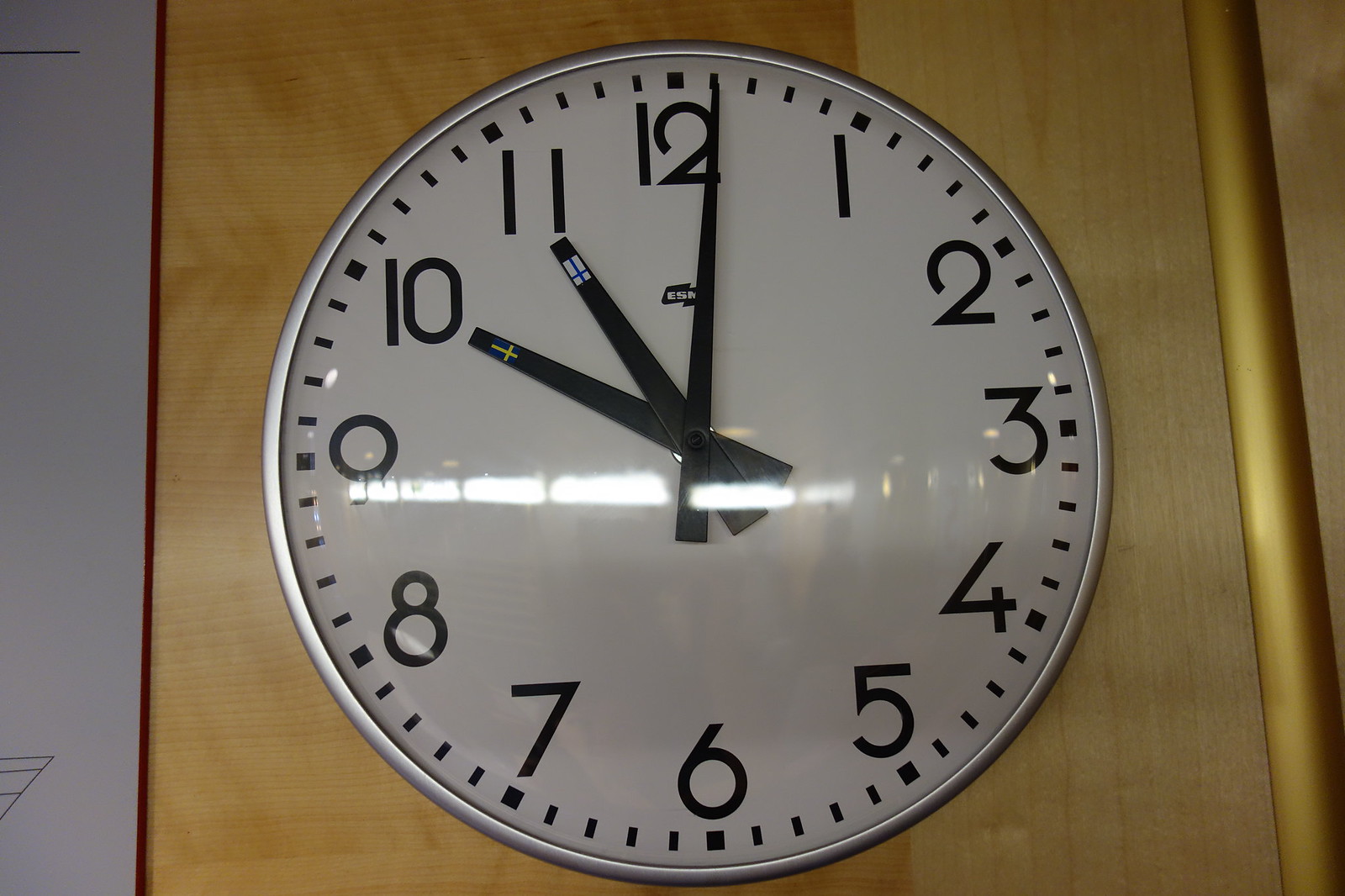This photograph captures a modern, simplistic clock hanging on a light wooden paneled wall, possibly in an office or classroom. The clock features a slightly reflective, narrow silver circular frame with an off-white face and large, black, loopy font numbers. It has three hands: an hour hand, a minute hand, and a longer second hand. Both the hour and minute hands are detailed with two distinct flags; one flag has a blue cross over a white background, and the other has a yellow cross. A manufacturer's mark, possibly reading "ESK," is centered just above the middle of the clock face. The background includes wood paneling with gold trim and a glare from low, narrow windows stretching across the space. To the left of the clock is a gray-colored poster frame.